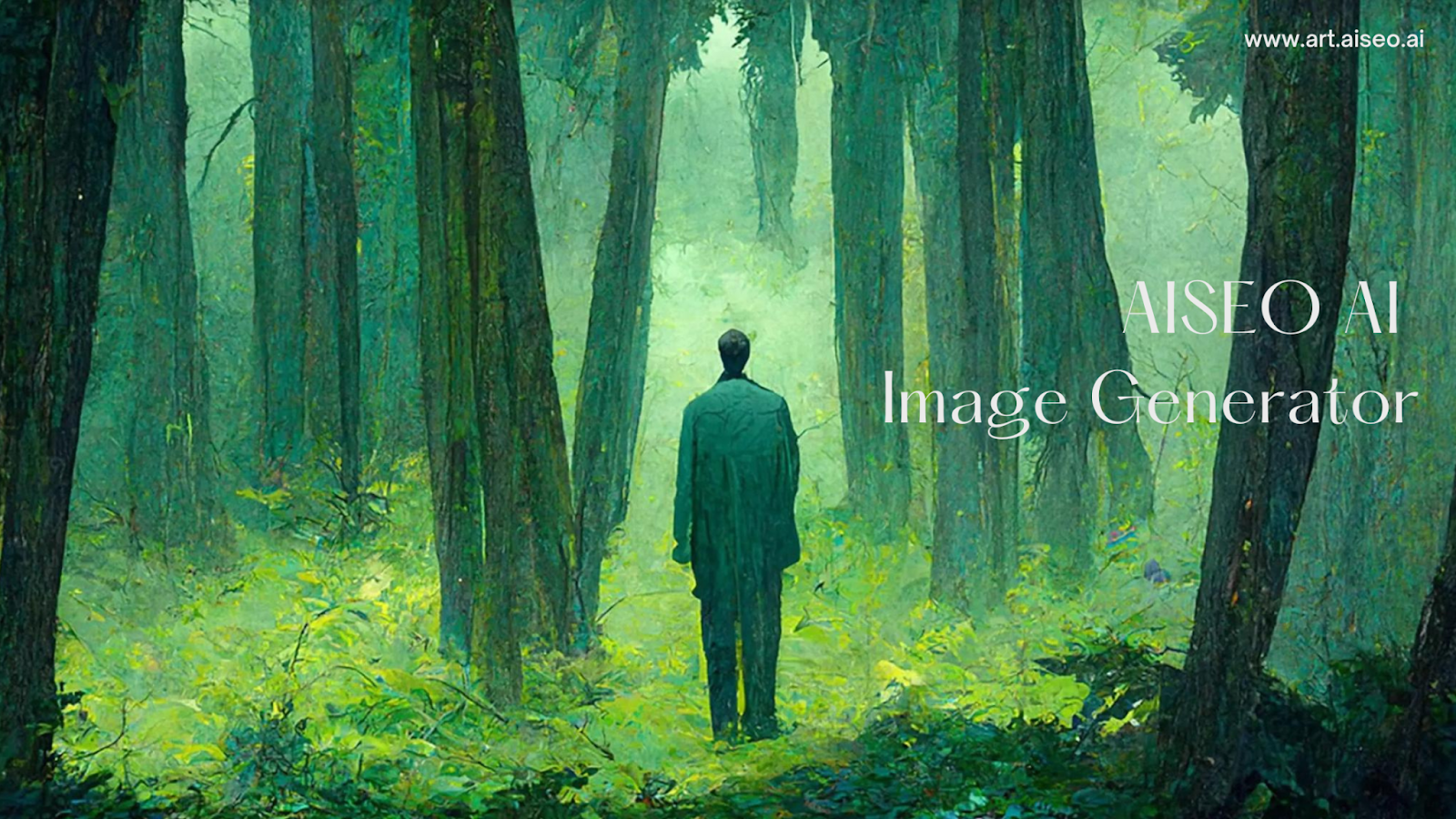This image, created by the AISEO AI image generator, displays a whimsical, cartoon-like forest scene. Dominating the image is a person in dark, bluish-green clothing, standing with their back to the viewer in a forest clearing. The person's short, dark hair is visible, and they wear a long coat and pants. The forest around them is filled with tall tree trunks that extend out of the frame, making the tree leaves and branches invisible. The trees vary in darker greenish-blue shades, providing a depth effect with nearer trunks appearing darker. The ground is covered with light green plants and undergrowth, depicted in an art style that reduces detailed elements. In the top right corner, white text reads "www.art.aiseo.ai," with "AISEO AI image generator" below it, both in clear, readable font.